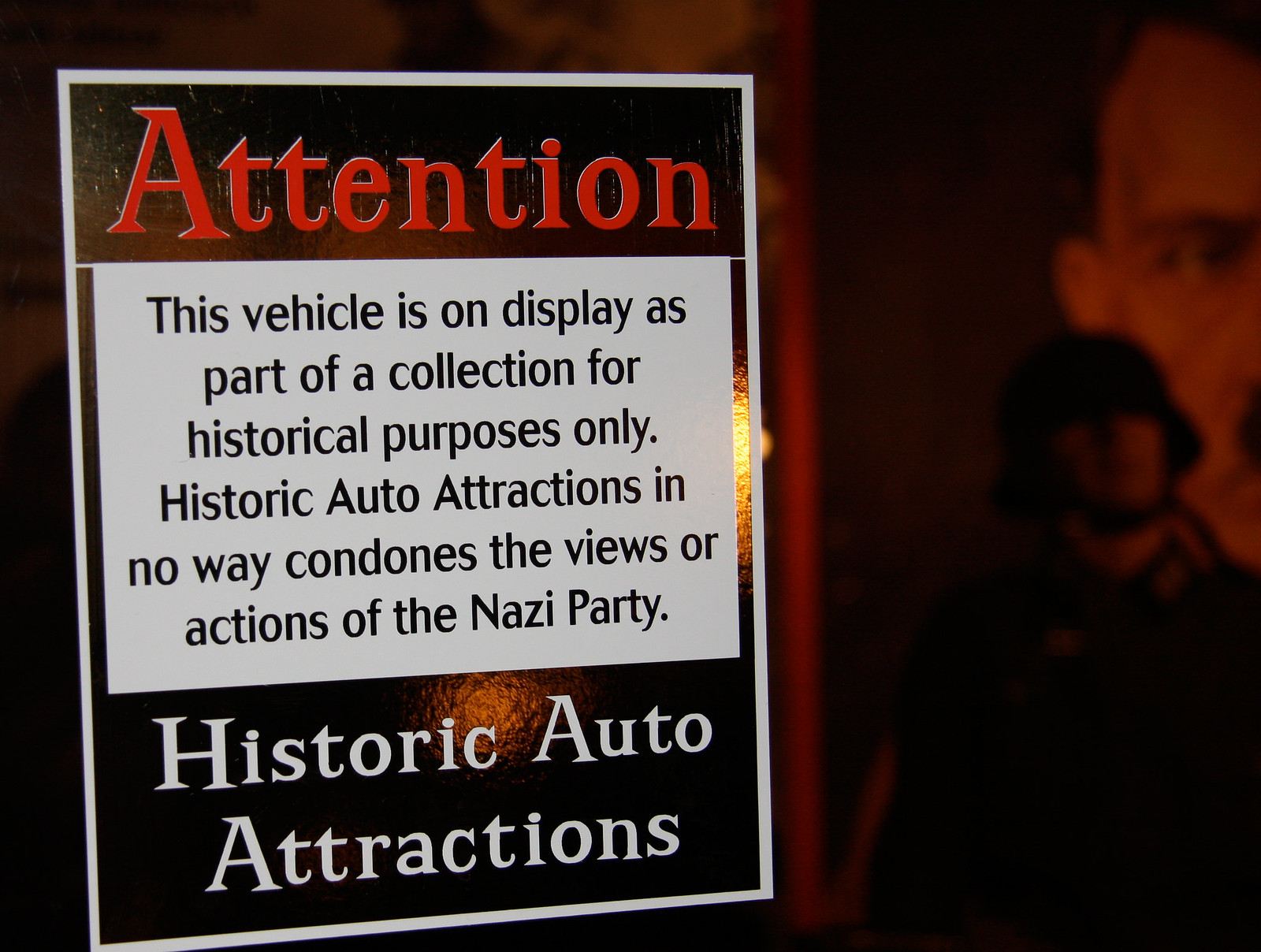The image depicts a slide in a dimly lit, dark red-hued room, primarily featuring a prominently displayed poster on the left side. The poster is bordered with white, containing a black background. At the top of the poster, bold red text reads "ATTENTION." Below, within a rectangular section, black ink states, "This vehicle is on display as part of a collection for historical purposes only. Historic Auto Attractions in no way condones the views or actions of the Nazi party." Beneath this in white font, "Historic Auto Attractions" is printed. The right side of the image showcases a shadowy figure resembling a soldier with a bucket hat and strap, partially obscured. In the background, you can discern a partially visible portrait of a man, possibly Adolf Hitler, his face cut off by the poster's edge, adding to the eerie atmosphere. Additionally, there appears to be an outline of a mannequin adorned in a Nazi costume near the bottom right corner. The overall scene is accentuated by the room's dark, red-tinted lighting, creating a somber and historic ambiance.